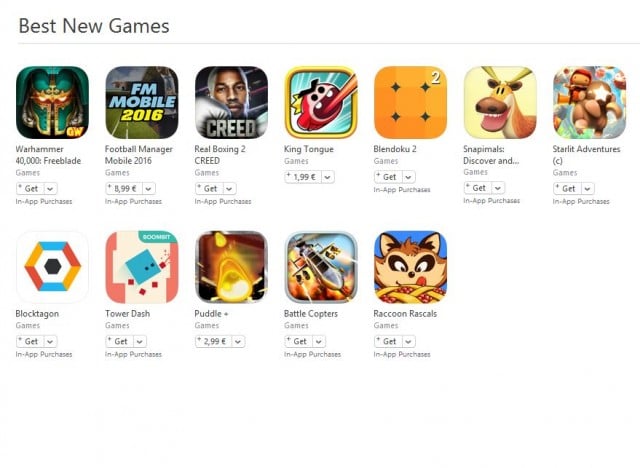**Detailed Caption:**

The image is a screenshot of a webpage showcasing various popular mobile video game applications under the prominent heading "Best New Games," displayed in bold at the top left corner. Below this header, a thin light gray line separates it from the content beneath. 

Two rows of game icons are presented in a grid format. The top row features seven square icons, while the bottom row comprises five. 

In the top left corner of the grid, there is an icon depicting a green and gold figure that resembles either a creature or a helmet. This icon belongs to "Warhammer 40,000: Freeblade." Directly beneath the icon, the name of the game is followed by the word "Games" and a blue "Get" button. An additional note indicates that the game includes in-app purchases.

Next to it, an icon resembling a racetrack catches the eye, which is actually a football field. This image represents "Football Manager Mobile 2016," priced at $8.99. A small note beneath the title indicates that in-app purchases are available.

To the right of the football game, there is an icon showing a black man wearing a silver boxing glove. This refers to "Real Boxing 2: Creed," with the word "Games" following the title. Below this, there is a "Get" button, indicating that the application can be downloaded for free, with the possibility of in-app purchases mentioned below.

All these icons are neatly arranged and suggest that these are downloadable video game applications, accessible for mobile phones or computers.